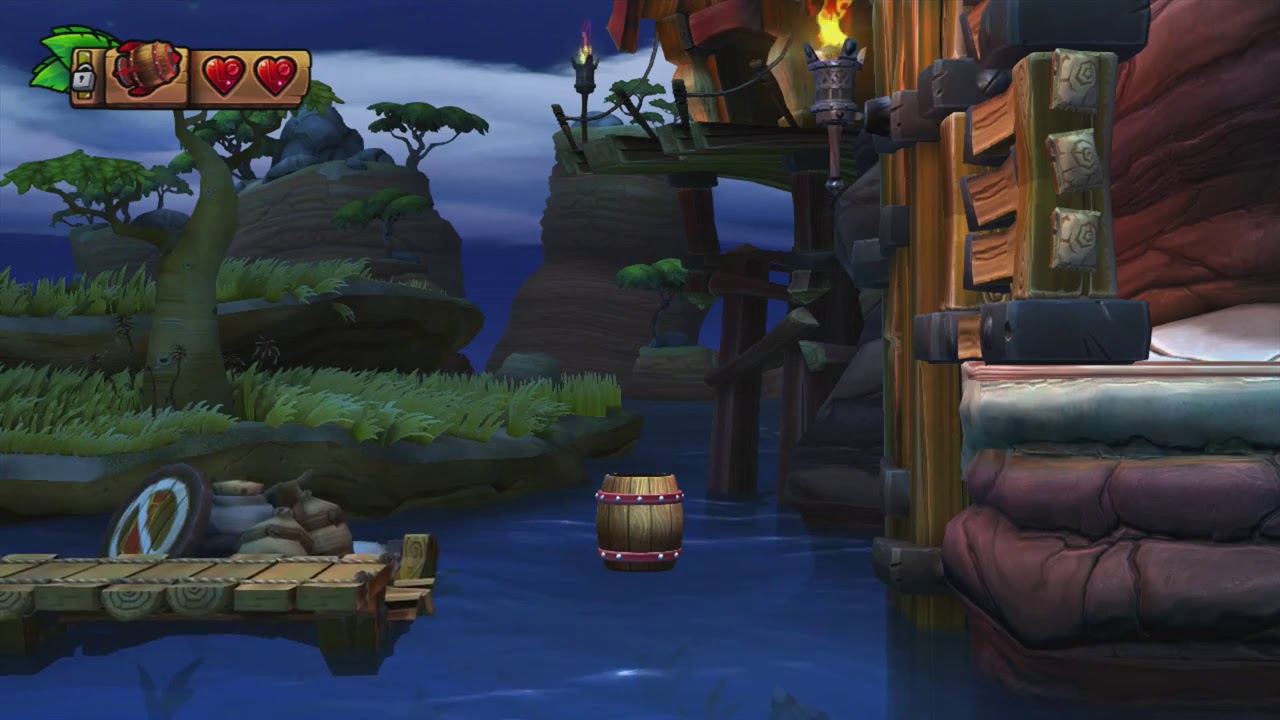This detailed video game screenshot shows a serene yet mysterious swamp or lake scene, dominated by a wooden and stone cabin resembling a small castle, positioned on the right side. The structure includes a drawbridge that's raised, preventing any entry. A torch glows warmly beside the door of the cabin. In the foreground, a wooden barrel floats on a body of water near the center bottom of the screen, drawing the viewer's attention. To the left, a wooden dock or pier constructed from half logs and planks extends into the water, held together with ropes.

Behind the dock, a small grassy island hosts a tree, and there are rocky formations with trees atop them scattered further in the background, creating an "Avatar-like" aesthetic. The scene is lit nicely with visible white clouds and a blue sky above.

In the upper left corner of the screen, there are several game interface icons: a health bar featuring two red hearts, an icon resembling a rocket ship, a padlock symbol, and graphics of green leaves, possibly representing some game mechanics. The overall color scheme features dark tones interspersed with natural elements and subtle details, including a mountain with a bridge and an open doorway leading to the cabin. The image conveys a blend of adventure and mystery, possibly from a game like Donkey Kong Country.